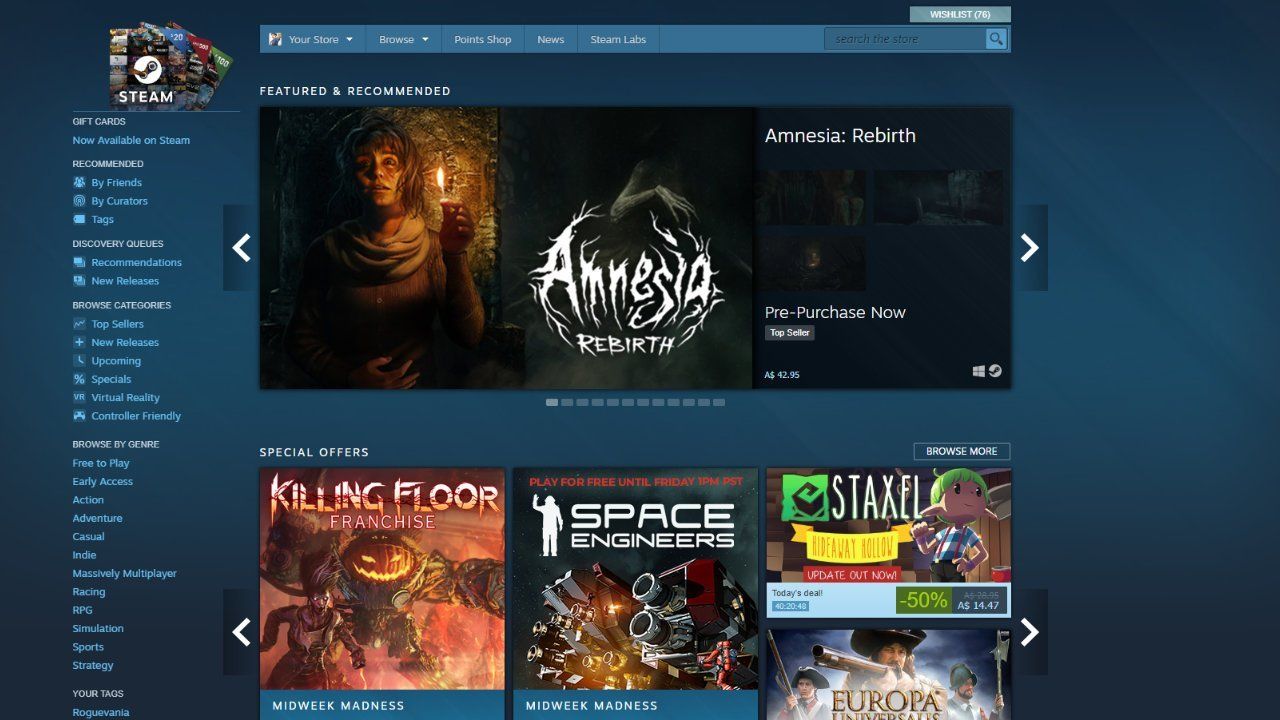A screenshot from the Steam gaming website prominently displays the "Featured & Recommended" section, highlighting the game "Amnesia: Rebirth." The cover art features a haunting image of one of the game's characters. It also includes a "Pre-purchase Now" option. Below this section, there is a "Special Offers" segment showcasing discounts on the "Killing Floor" franchise, adorned with themed graphics such as a pumpkin and a witch or monster, as well as another offer on "Space Engineers," represented by an image of a spaceship. The top area of the website, beneath the Steam logo, includes various navigational links that are too small to discern in detail. Additional advertisements for other games are visible towards the bottom.